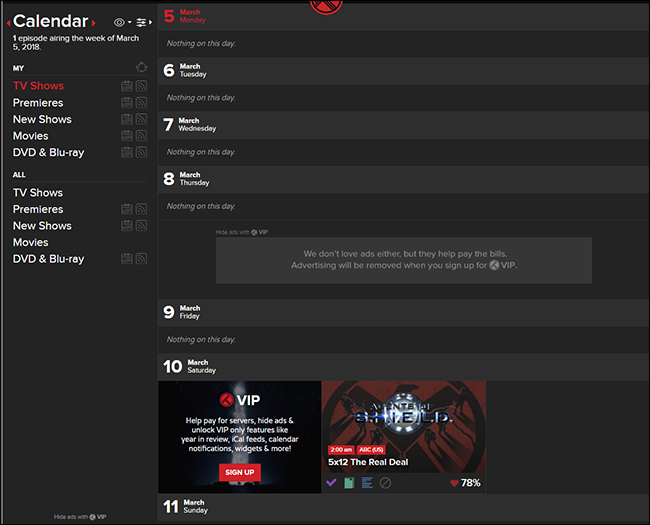The image depicts a detailed interface of a digital calendar with a predominantly black background accented by white text and gray highlights. At the top left corner, there's a column header labeled "Calendar." Flanking this header are red arrows pointing left and right. Next to these arrows is an eyeball icon with a downward arrow, followed by a filter graphic with an arrow pointing to the right. The header also includes text indicating, "One episode airing the week of March 5th, 2018."

Below this header, there are two sections. On the left, one section, labeled "My TV Shows" in a combination of red and white text, includes categories such as premieres, new shows, movies, DVD, and Blu-ray, each with corresponding icons to the right. Adjacent to it is another section labeled "All," containing similar categories.

The larger right-hand section is a detailed calendar view. The date "March 5th" is highlighted in red, noting no events for that day. Subsequent dates including March 6th and 7th are listed with no entries. On March 8th, it again states "Nothing on this day," followed by a gray advertisement mentioning, "We don't love ads either, but they help pay the bills. Advertising will be removed when you sign up for VIP." March 9th follows with no listings, and on March 10th, there are two advertisements. One includes a VIP sign-up prompt in a red box.

To the right, a SHIELD graphic logo is featured prominently. The logo consists of an eagle on a red background, with the acronym "SHIELD" in a police-like font colored in black and blue. In the lower right corner, a red heart icon with white text indicates a rating of 78%.